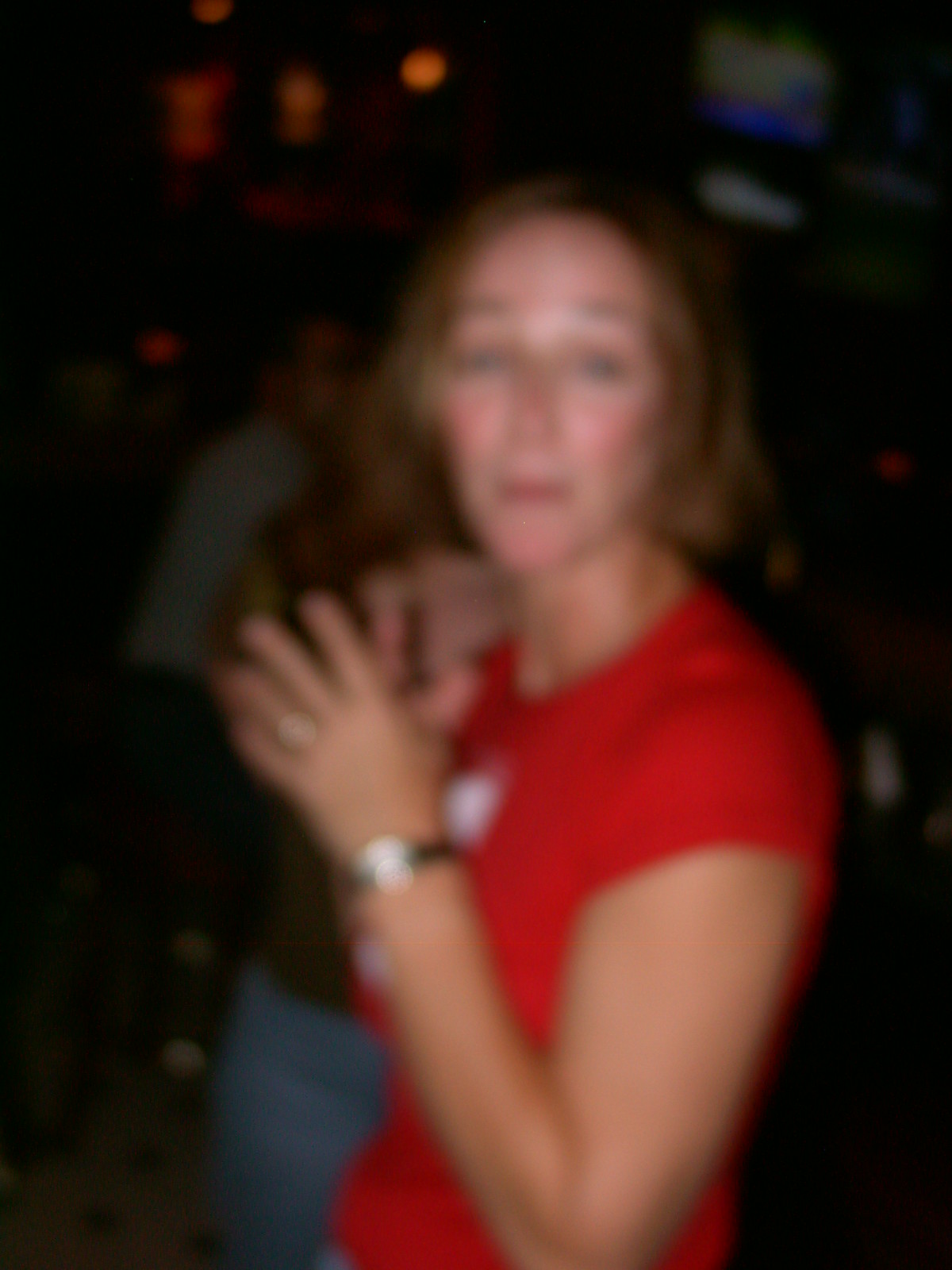In the photograph, the main focal point is a woman dressed in a red short-sleeve shirt and a black wristwatch. She also has a ring on one of her fingers. Her hair is short and a blend of brown and blond shades. In the background, there are other people visible; one person is wearing a green shirt and jeans, while another is wearing a white shirt. Above the woman's head, there is a television that appears to be turned on. The floor shows a hint of white and black tiles. The image is quite blurry, but in the background, some lights and darker wood tones are visible.